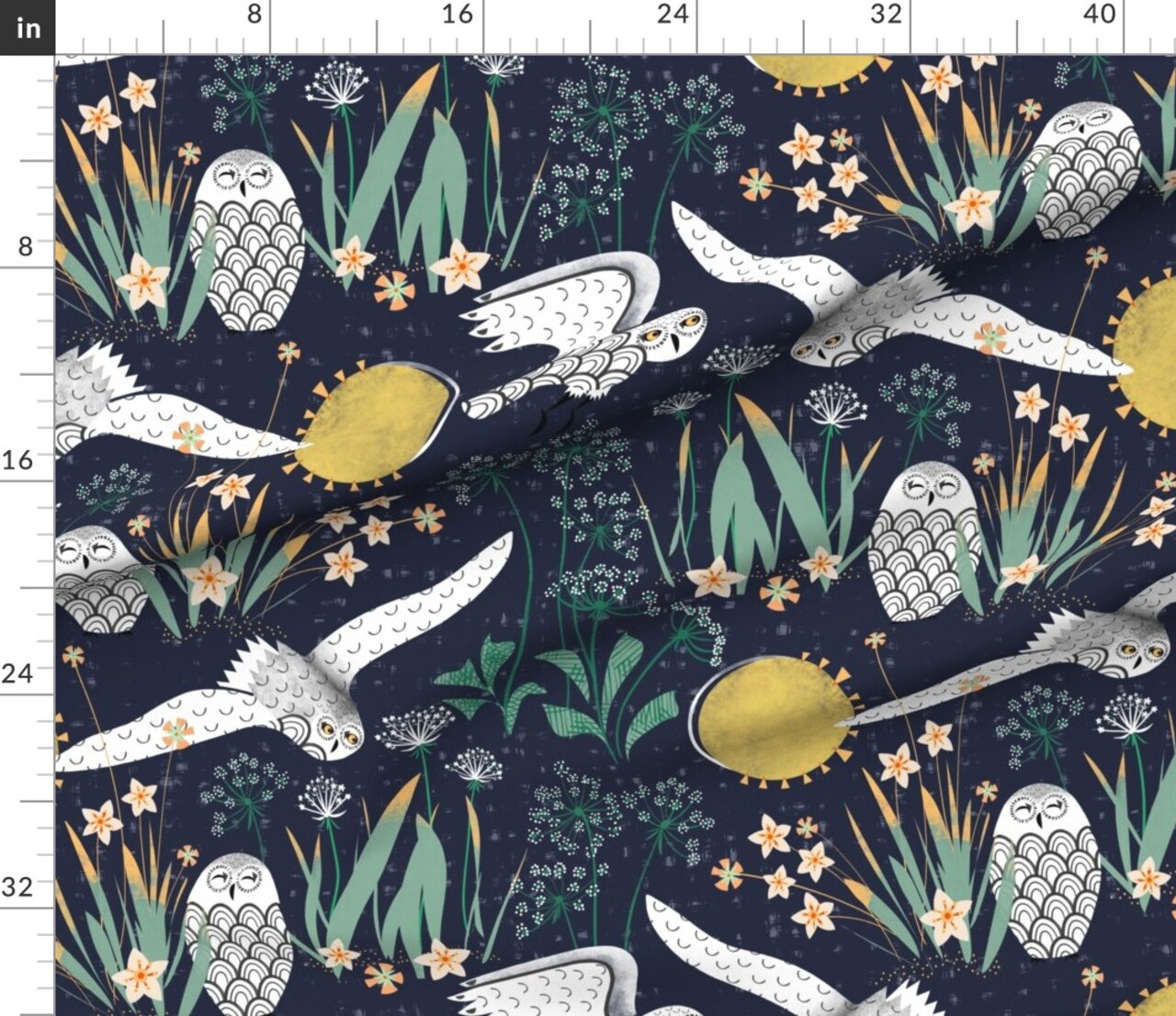This is a color photograph of a dark, black fabric, possibly laminate paper or a type of tapestry, adorned with images of owls and floral patterns. The fabric, set against a backdrop of a measuring grid that prominently features rulers along both the vertical and horizontal axes, is marked in intervals of 8 inches, reaching up to 40 inches and beyond. The design showcases a variety of modern, contemporary-style owls depicted in different poses—some perched, some in flight, and others in unique, side-profile angles. One particular owl, with its wings spread wide, evokes an angelic appearance. Interwoven amongst the owls are diverse, colorful flowers that are predominantly orange and white, along with intricately illustrated plants. Adding to the whimsical nature of the design, there are repetitive images of suns scattered across the fabric, further enhancing its artistic and stylized appeal.